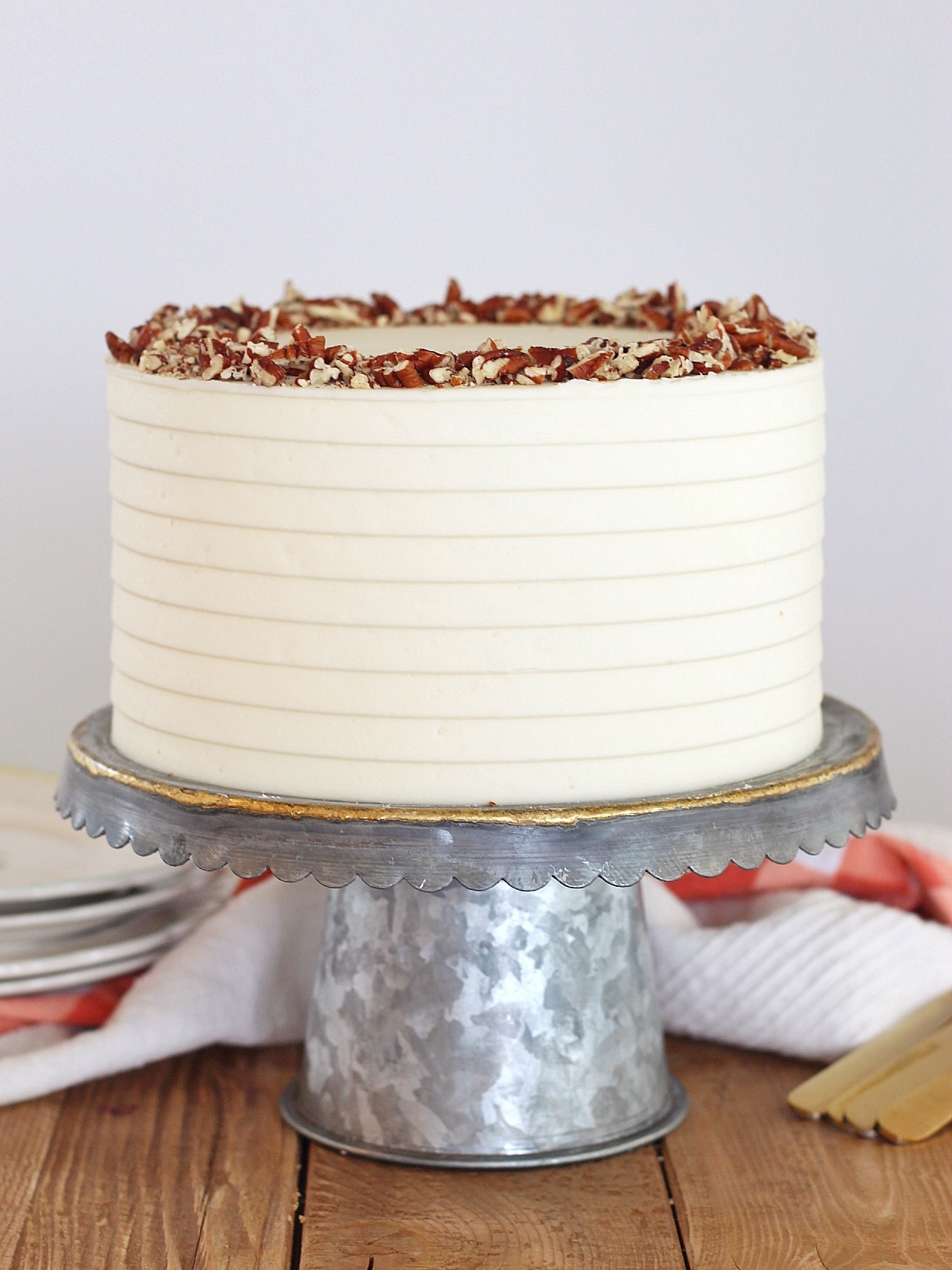In the image, a metallic cake tray, adorned with gold trim, sits on a brown wooden table against a light lilac background that fades into gray from top to bottom. The centerpiece, a nine-layered white cake, is perched on the tray, its frosting arranged in straight lines that suggest neat, distinct layers. The top of the cake is decorated with a circular pattern of ground nuts, likely walnuts or almonds, although the distribution appears haphazard. Behind the cake, a white cloth has been casually pushed back, while the lower left side of the table features a collection of plates. To the right, a set of small wooden utensils, possibly spoon handles, are arranged. The cake holder itself shows signs of wear, with some corrosion visible around the edges.